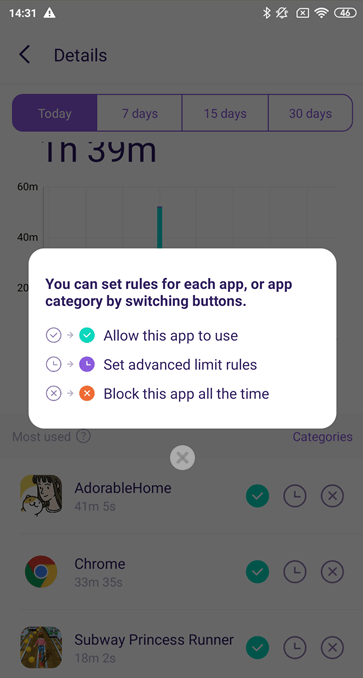Caption:

"A screenshot of a user interface from a mobile application displays a dialogue box with various settings options. At the top, the box instructs users, 'You can set rules for each app or app category by switching buttons.' Below this, the interface showcases three different buttons and their corresponding functionalities: 

1. A checkmark button indicating 'Allow this app to use,' transitioning to a highlighted neon version of the same button.
2. A timer button labeled 'Set advanced limit rules,' accompanied by an arrow pointing to a purple-filled version of the button.
3. An 'X' button reading 'Block this app all the time,' pointing to an orange-filled version of the button. 

An additional 'X' is located at the bottom of the dialogue box, presumably to close the settings menu."